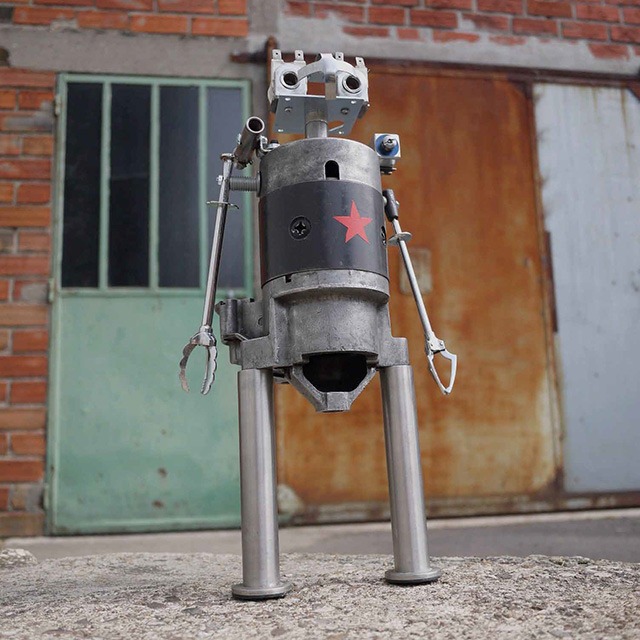The image features a small, intricately crafted robot sculpture standing on a gray, stone-like ground. The robot has a barrel-shaped torso adorned with a black stripe and a prominent red five-pointed star. Its stainless steel legs are attached to the torso with visible bolt sections, resembling components from an old electrical starter. The robot's arms, extending outwards, end in graspable claw-like appendages made of metal rods and clamps, and its head features two hole-like eyes atop a structure resembling a neck pipe.

In the background, an oxidized copper-green door with four vertical window panes and green hinges is visible. Adjacent to this green door is a rusted metal door panel, followed by a section of a white wall. Above the doorways, the building's facade transitions from granite blocks to red bricks, with the bricks on the left side appearing more brownish-red than the reddish bricks directly above the doorway. The overall scene gives an ambiance of an old, weathered structure, providing a stark contrast to the shiny metal complexity of the robot in the foreground.